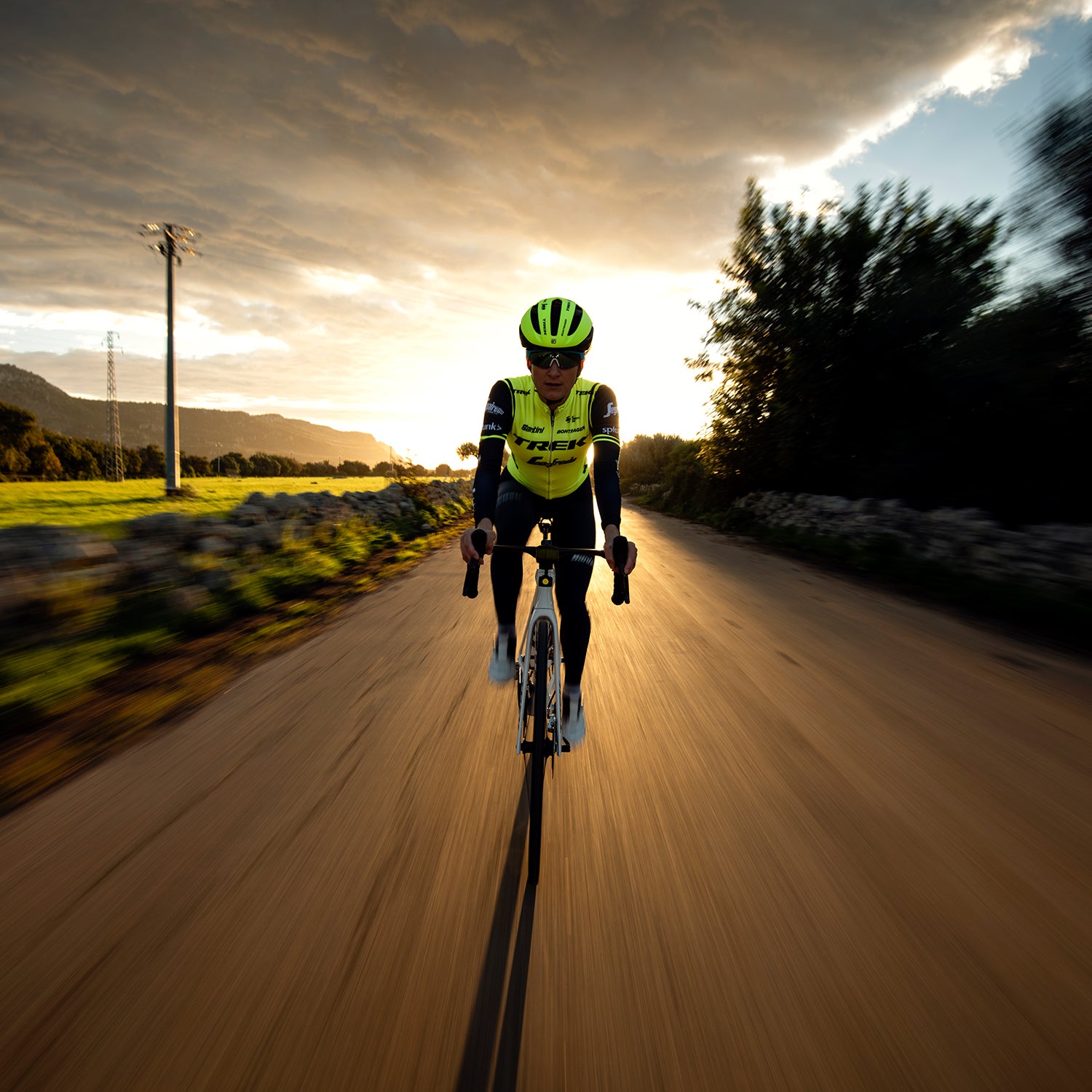A professional cyclist, dressed in a neon greenish-yellow jersey with black sleeves and black leggings, races towards the camera on a white bike with black handlebars. Adorned with a matching neon helmet and black sunglasses, the cyclist's white shoes blur slightly, capturing the velocity of the ride. The background appears in motion with the slightly blurred effect, enhancing the dynamic feel of the image. Surrounding the cyclist, the landscape features a mixture of elements: open green fields with a prominent telephone pole on the left, a stone wall and bushes to the right, and some visible hills in the distance. The sky above is grey with clouds, but glimpses of blue sky and the sun breaking through give a dramatic contrast, suggesting either dawn or dusk. The scene is captured on a grey road, adding to the overall impression of speed and motion.